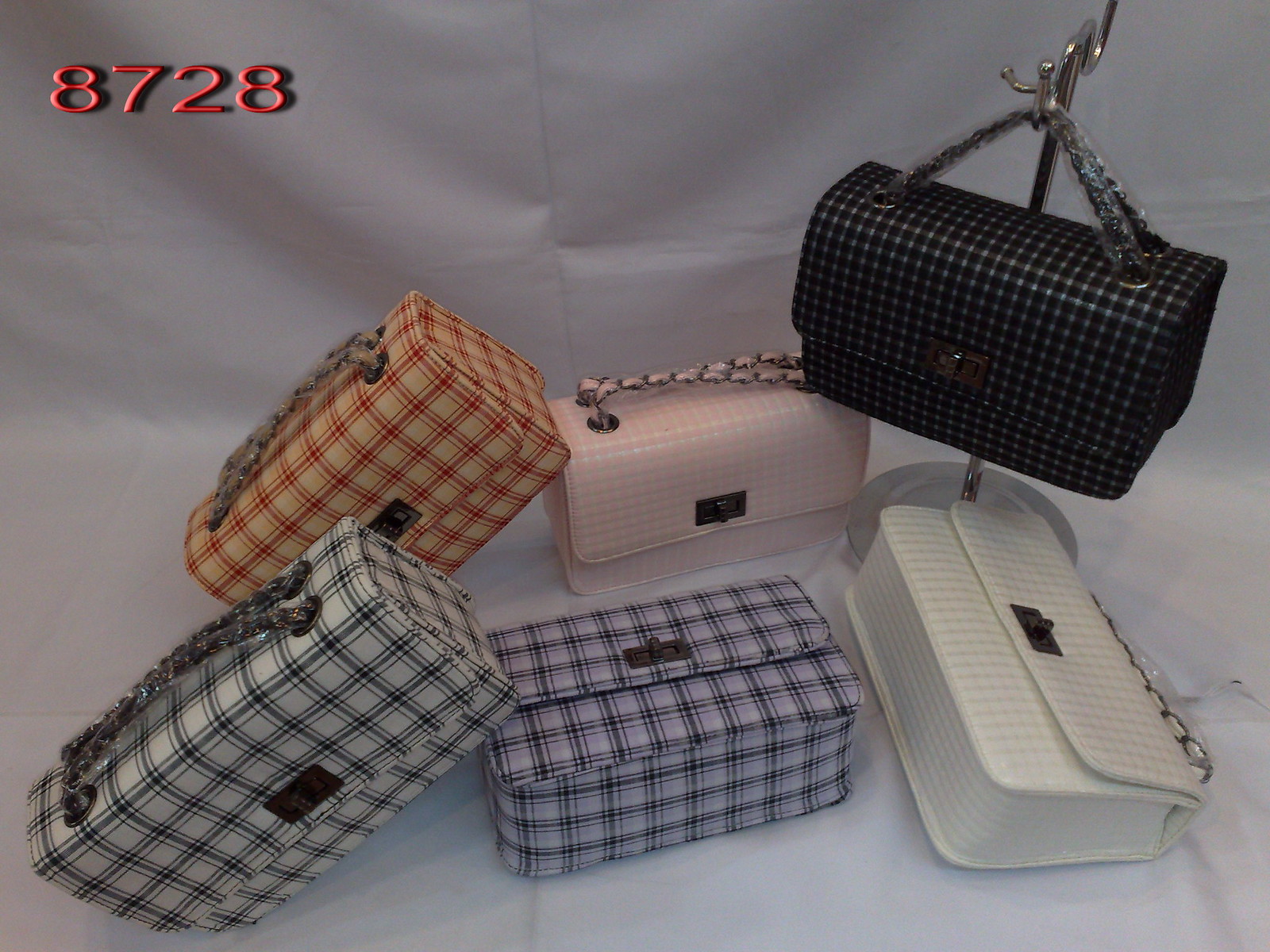The image showcases a display of six small, rectangular handbags arranged on a wrinkled white paper background. In the upper left corner of the photo, the number "8728" is prominently displayed in red, possibly indicating a product code. 

In the back row, starting from the left, there is an orange and red plaid handbag beside a plain pink handbag. To the right of the pink handbag is another plaid handbag, this one featuring a black and gray checkered pattern. The front row presents three more handbags: on the left is a green and blue plaid bag, next to it is a handbag with white, purple, and blue shades, and on the far right is a plain white handbag with a black clamp on the outside. 

Notably, one of the black handbags is hanging on a chrome pole with a hook, suggesting that this display might be in a shop window or used for listing the products in a sales picture. The handbags share a similar boxy shape with short handles, reminiscent of toiletry bags or construction worker's lunch pails, emphasizing their practical yet possibly high-fashion appeal.